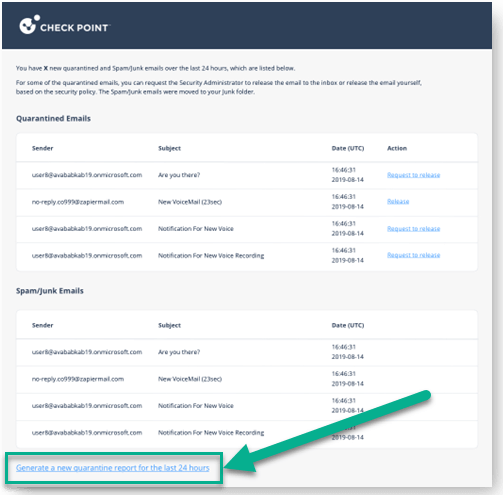The image is a screen capture of an online application window with a white background. A black horizontal bar lines the top of the window. A subtle 3D shadow effect is present on the right side and bottom edge of the window, giving it a slightly elevated appearance. The text within the window is generally small and blurry, making it hard to decipher specific words. However, on the left side, clear and bold black text reads "Guaranteed Emails" and "Quarantined Emails." Beneath these titles are about four to five rows of indistinguishable small text. Further down, another section, again in bold black text, reads "Spam/Junk Emails," followed by another five rows of hard-to-read text. At the bottom left corner, a highlighted green rectangular box stands out, accompanied by a long green arrow pointing toward the text box, emphasizing it.